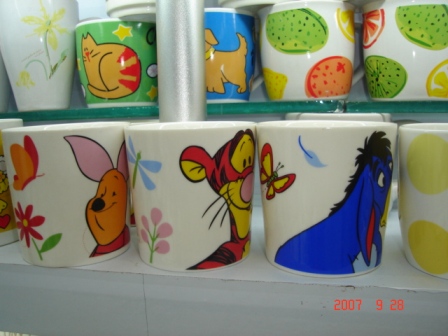This photograph, dated September 28th, 2007, showcases an assortment of colorful mugs, each with unique and detailed designs. In the bottom right corner of the image, the date is digitally imprinted in red text. The collection features ten mugs, divided into two rows. The top row includes five mugs, starting from the left: a white mug adorned with yellow flowers, followed by a green mug featuring an orange cat with darker orange stripes against a green background, and then a blue mug with a brown dog on it. The last two mugs on this row are white, each decorated with vibrant images of orange oranges, green limes, and yellow lemons.

The bottom row also displays five mugs, all predominantly white and themed with characters from Winnie the Pooh. Starting from the left: the first mug features Piglet, accompanied by an orange-red butterfly, a red flower with a green leaf, and additional small plants. The next mug showcases Tigger, with his orange and yellow fur and black stripes, also accompanied by a blue-winged dragonfly and a small pink flower. Completing the character trio is Eeyore, depicted in blue with pink inside his ears and a black mane, alongside an orange and yellow butterfly. All mugs are meticulously designed, primarily with children's cartoon themes and some with colorful fruit motifs, creating a vibrant and cheerful collection.